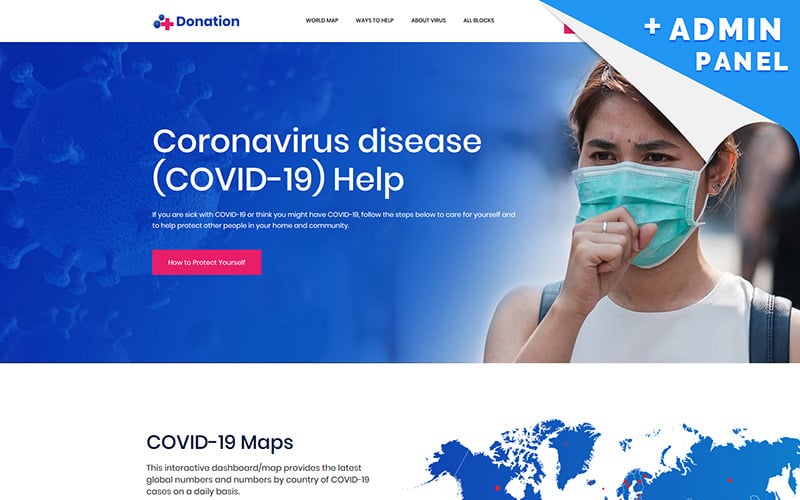The image depicts a detailed webpage layout related to COVID-19 information. 

**Header**: Located at the top left, features text labels such as "World Map," "Ways to Help," "About Virus," and "All Blogs."

**Donation Section**: Positioned prominently with the word "Donation" in blue text alongside a red plus sign and two blue dots, all set against a white background.

**Right Side**: A visually appealing effect shows the page peeling back from the top right to the bottom, unveiling an admin panel. The revealed background is blue with the words "Plus Admin Panel" written in white.

**Central Section**: Dominated by an informative space featuring a coronavirus image background with white text. The key message reads: "Coronavirus Disease COVID-19 Help. If you are sick with COVID-19 or think you might have COVID-19, follow these steps below to care for yourself and to help protect other people in your home and community." Below this, a red button labeled "How to Protect Yourself" stands out prominently.

**Right Side Image**: Displays a woman coughing, wearing a face mask, a ring on her middle finger, a blue backpack, and a white vest. 

**Bottom Section**: Features a white background with text on the left side that says, "COVID-19 Maps. This interactive dashboard or map provides the latest global numbers and numbers by kind of COVID-19 cases on a daily basis."

**Bottom Right Corner**: Shows a map in blue and white with red dots indicating COVID-19 cases in various countries.